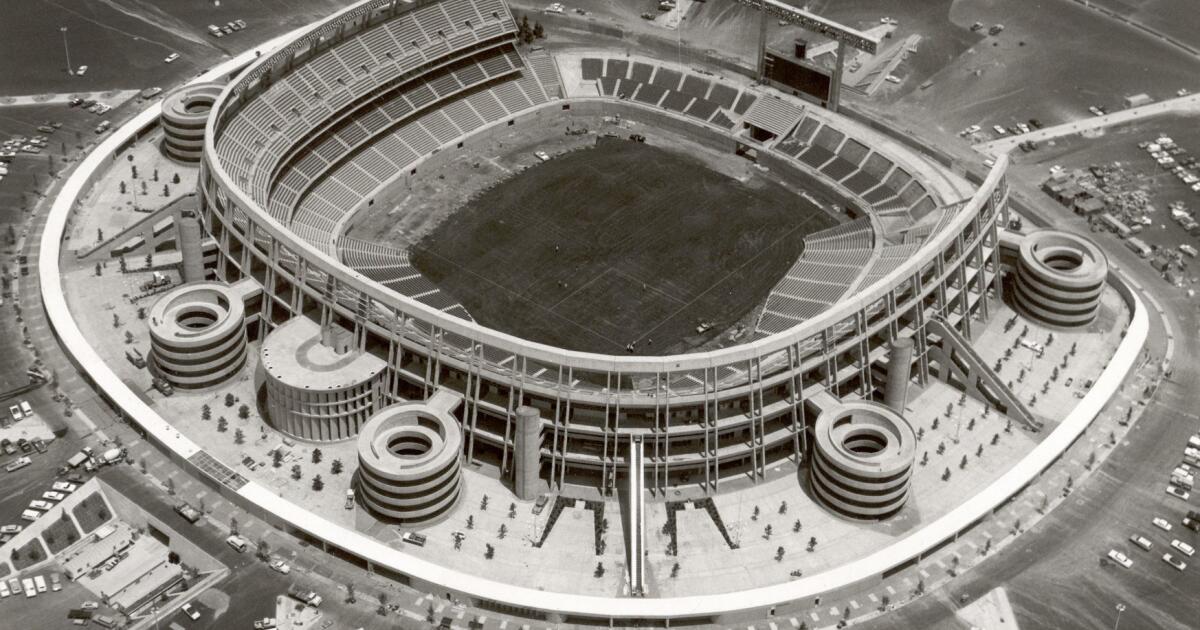This black-and-white aerial photograph captures a large, circular sports stadium, possibly a football or baseball stadium, surrounded by parking lots and small trees, indicative of a period ranging from the 1960s to the 1990s. The image shows the entirety of the stadium from a significant distance, revealing empty bleachers and a field that may not be fully developed. The field inside the stadium appears green, suggesting it is grass, but no people are visible either on the field or in the stands. Around the stadium, there are multiple scattered cars in the parking lots, which are not densely packed. The outer structure of the stadium features five distinct circular attachments, possibly for entryways. The stadium also has a spiral design with alternating light gray and black tones. The scene evokes an older, somewhat deserted atmosphere with its lack of activity and scattered vehicles in the surrounding lots.